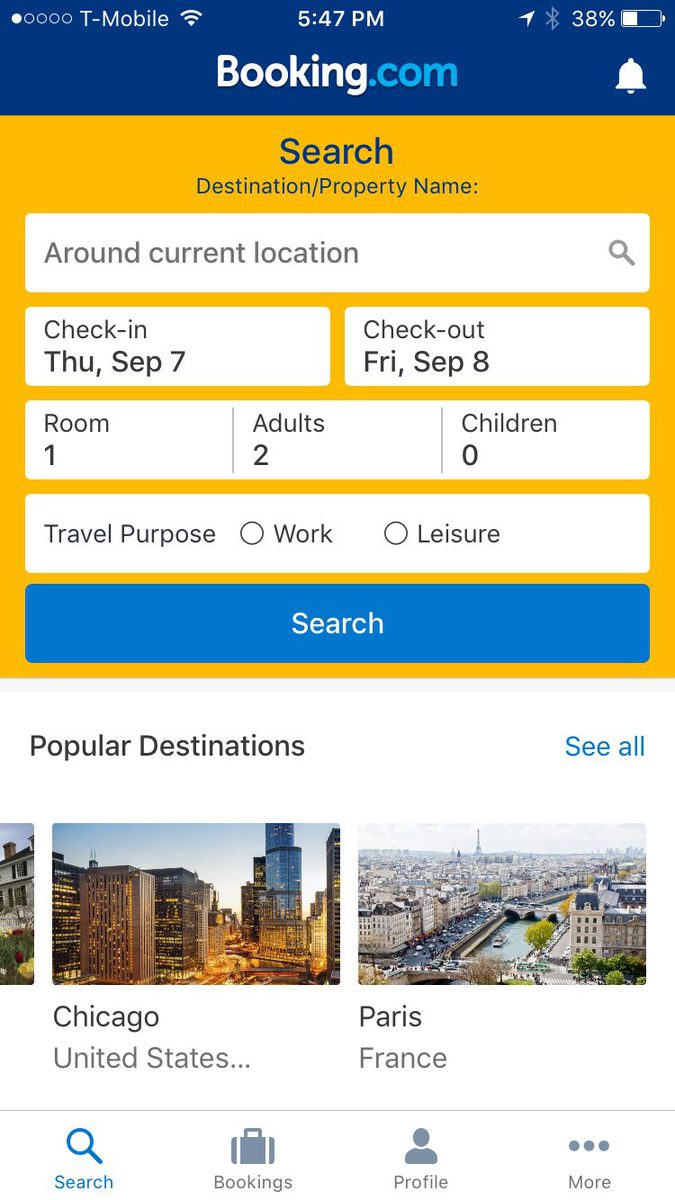The image showcases the user interface of the Booking.com mobile app on an iPhone. The phone displays 1 out of 5 signal bars with T-Mobile as the carrier, and the time is 5:47 PM. Location services and Bluetooth are enabled, with the battery level at 38%. 

The headline reads "booking.com" with a notification icon to its right. Below is a prominent search bar labeled "Destination/property name," inviting users to input their destination or property of interest. 

The next section pertains to reservation details. The check-in date is set for Thursday, September 7th, and the check-out date for Friday, September 8th. The search parameters include one room, two adults, and zero children."

The options for the purpose of travel, "Work" and "Leisure," are available but not selected. A blue "Search" button allows users to proceed with their specified search criteria.

Popular destinations listed include Chicago, United States, and Paris, France, among others not visible in the image. The bottom menu bar offers navigation options: Search, Bookings, Profile, and More, represented by three dots.